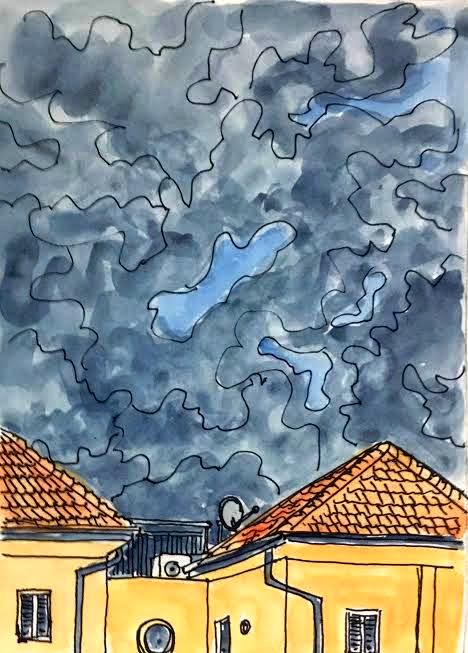This captivating watercolor painting showcases a serene urban scene characterized by an array of low, adobe-style buildings. The structures, painted in a warm, light brown hue, feature visible windows, eave troughs, and distinctive brown tile roofs converging to sharp points. Dominating the nuanced skyline is a nearly monochromatic gray sky adorned with a jigsaw puzzle pattern of clouds, some of which are fragmented enough to reveal patches of blue. Notable rooftop details include an air conditioning unit centrally placed, an upward-pointing satellite dish, and a cage-like structure silhouetted against the horizon, adding intriguing elements to the tranquil setting.